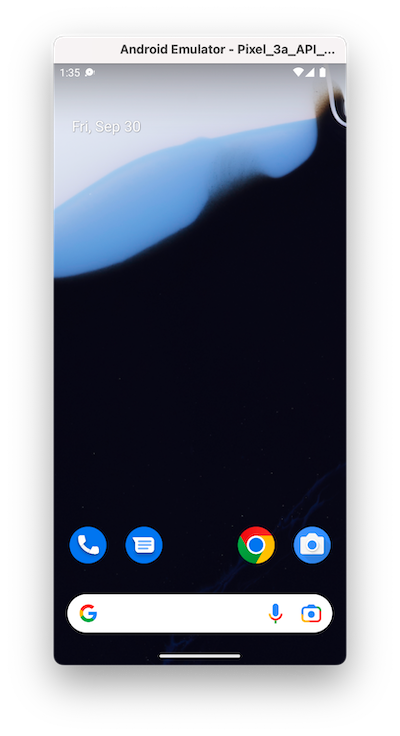This image is a detailed screenshot of a cell phone interface displayed on an Android Emulator running the "Pixel_3A_API..." configuration. The top of the screen features a light gray banner with black text reading "Android Emulator - Pixel_3A_API..." The status icons on the right of this banner show the battery level, Wi-Fi connection, and cell signal strength, all set against a gray background. Below the banner, the screen transitions from light gray to powder blue, which slopes upwards to the right. The lower portion of the screen displays a black background, which arches up in the center and goes past the powder blue section.

In the middle of the screen, there's a row of circular icons: the first blue circle contains a phone icon, the second blue circle contains a chat icon, the third icon is a Google Chrome logo, and the fourth blue circle contains a camera icon. Just above these icons, there is a white search bar labeled "Google," featuring a small microphone icon on the right and a camera icon within the search bar.